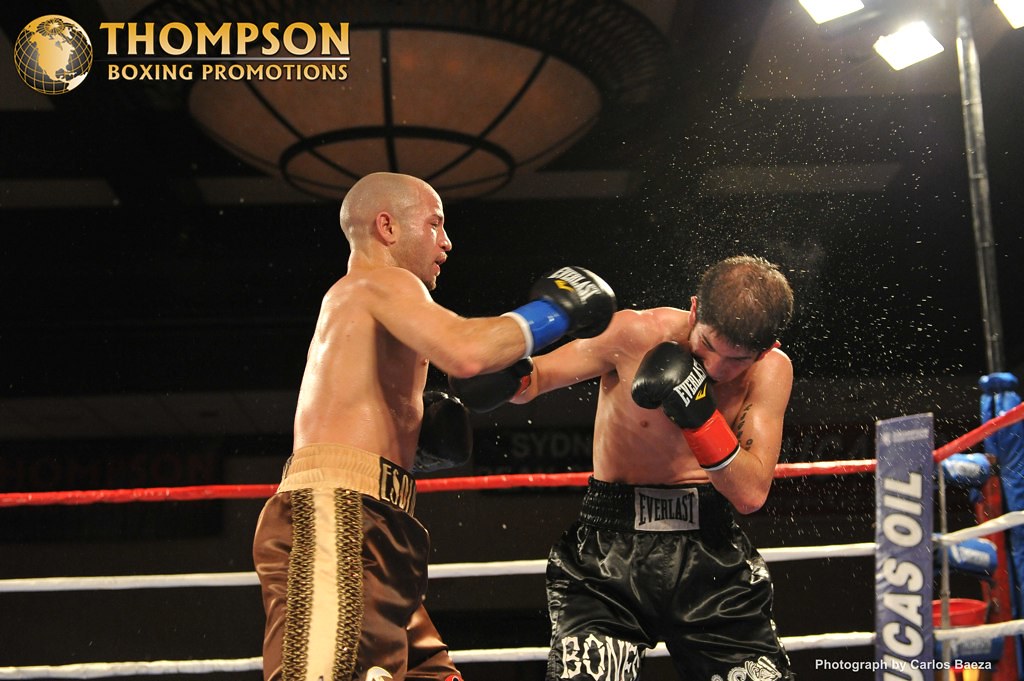The image captures an intense moment in a boxing match. In the center of the ring, two fighters engage in a heated exchange. The fighter on the left, wearing brown trunks with gold trim, throws a powerful punch towards his opponent. His gloves are a striking combination of blue and black. On the right, the opposing fighter, clad in shiny black Everlast shorts emblazoned with "Bones," reels from the impact, sweat dramatically spraying from his head. Both fighters' gloves are prominently featured, adding to the visual intensity of the scene.

The boxing ring is framed by ropes, with the top rope being red and the middle and bottom ropes stark white. Above the ring, lights illuminate the competitors, highlighting every detail of their struggle. In the upper left corner of the image, the logo for Thompson Boxing Promotions is displayed, featuring a globe beside the text. Adding to the arena's ambiance, a vertical blue sign reading "Lucas Oil" is partially visible in one corner. The overall setting is a showcase of athletic prowess and the raw emotion of the sport.